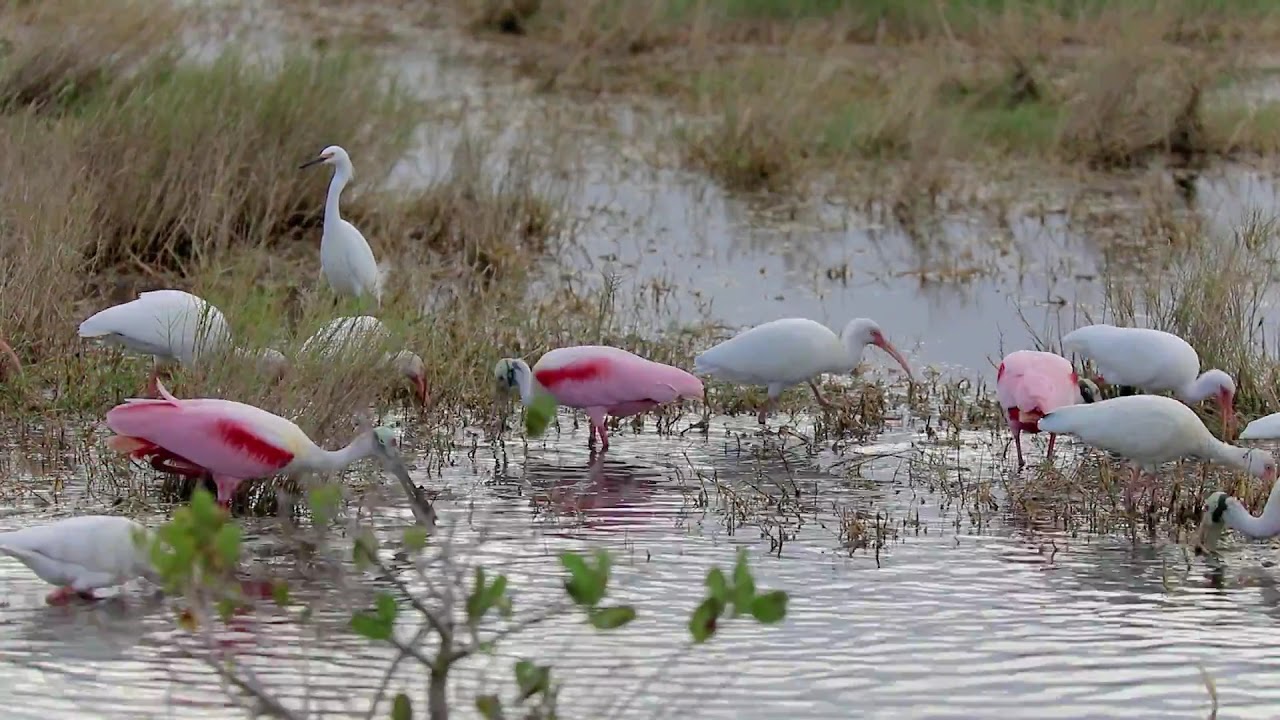This daytime image captures a serene scene of about ten birds in a shallow, swampy marsh. The water around them is dark and murky with patches of tan and green grass peeking through. Most of the birds are white, while three of them exhibit a pale pink hue with vivid, reddish-pink feathers on their wings. They possess long beaks and necks; most are bent over, seemingly pecking and searching for food beneath the water's surface. However, one bird stands out in the top left area of the image, standing upright amid its hunched companions. The water, only reaching up to their legs, is shallow and dotted with small shrubs and taller grasses in the background. The scene appears to be under a cloudy sky, casting a soft, diffused light over the tranquil marsh as the birds forage for their meal.